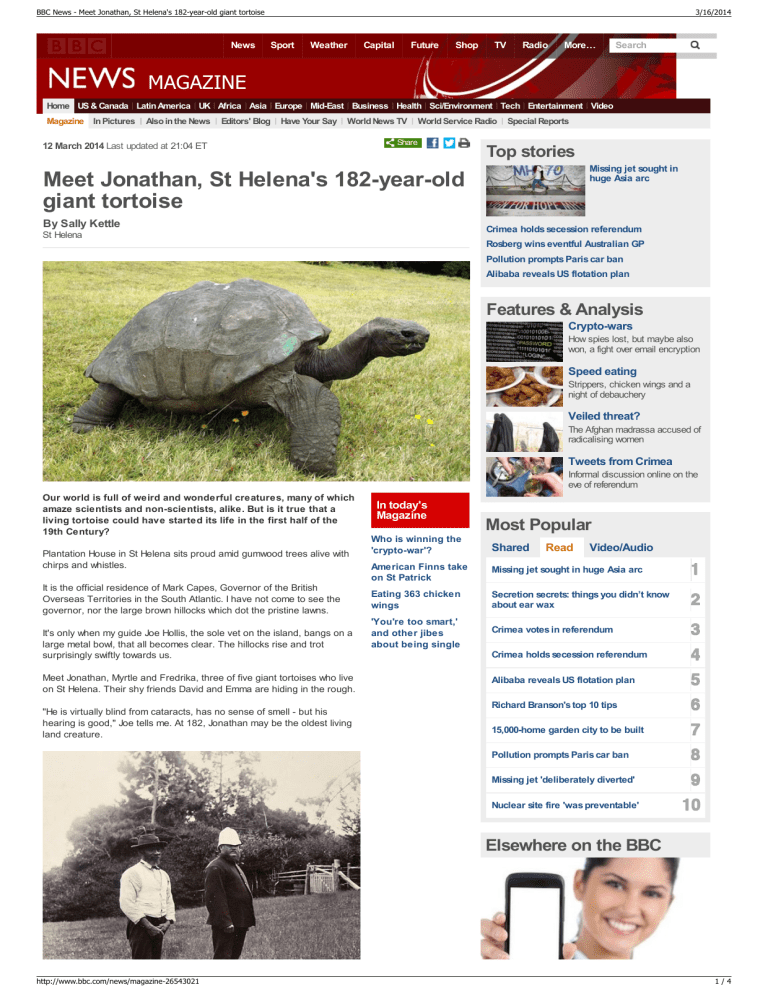In this image of a news article titled "Ms. Jonathan: St. Helena's 182-Year-Old Giant Tortoise," the layout features a detailed design characteristic of the PPC News magazine. The top left corner prominently displays the PPC News logo, while on the right, a red background showcases multiple tabbed sections including news, sports, weather, capital, future, shop, TV, radio, and more. Below this, another row of tabs provides navigation to various global regions and categories such as home, US, Canada, Latin America, UK, Africa, Asia, Europe, Middle East, business, health, social, environment, tech, entertainment, video, and special reports.

The main body of the article, dated 12th March 2014 with a last update on 21st April 2018, delves into the life of Jonathan, a giant tortoise residing on St. Helena. Written by Sally Kittle, the piece is accompanied by a vivid image of Jonathan, a black-shelled tortoise resting on green grass. The article is set against a crisp web page layout and begins by marveling at the diverse and unique creatures our world harbors, focusing on the remarkable fact that Jonathan could have been born in the early 19th century.

Describing St. Helena's Plantation House, the official residence of the island's governor, the narrative continues with the encounter of Joe Hills, the island’s sole veterinarian. Hills demonstrates how the tortoises, including Jonathan, Maitreyi, and Rodericka, respond to the clang of a metal bowl. Jonathan, despite being blind from cataracts and having no sense of smell, retains acute hearing and is believed to be the oldest living land creature at 182 years old.

The right sidebar of the article features a section labeled "Top Stories," listing headlines such as "Missing Giant Sword in Huge Asia," "Crime Hold Detective’s Blurry," "Future Analysis," "Crypt Wars," "Speed Eating," "Veiled Treat," and "Short Tweet from Crime A." The "Most Popular" section includes articles like "Secret Things You Didn’t Know About EOX," "Crime A Vote-In Referendum," "Alibaba Reveals U.S. Rotation Plan," "Richard Branson’s Top 10 Tips," "15,000 Home Guardian City to Be Built," "Population Prompt Perish," and "Nuclear Site Fire Was Preventable."

This vivid description encapsulates both the content and the layout of the news article, providing a comprehensive snapshot of the story and its surroundings.